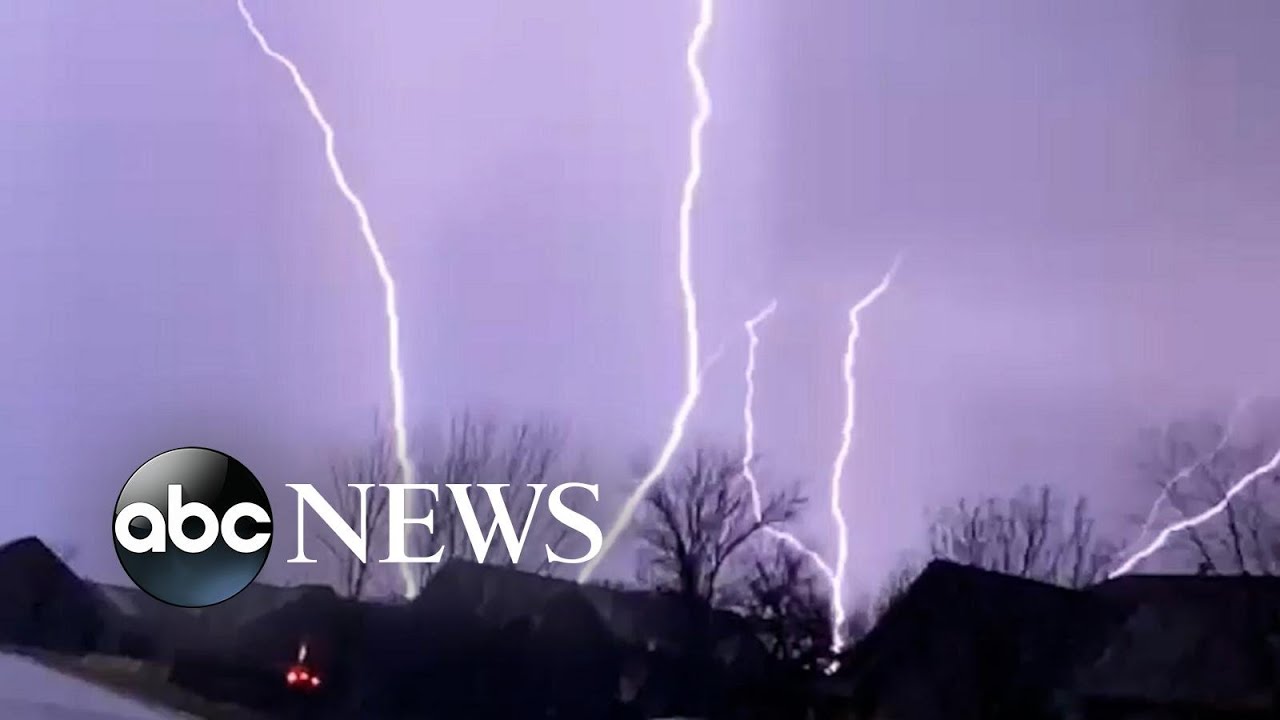This detailed image, likely a screenshot from a televised broadcast on ABC News, captures the ferocity of an outdoor thunderstorm in full color. The scene unfolds under a dramatic purplish-gray sky, filled with multiple lightning bolts striking in at least four different locations. The horizontal, landscape-oriented image focuses on a residential area enveloped in darkness, with silhouettes of several houses and numerous bare-branched trees at the bottom. There's a noticeable home with lights on at the bottom left, adding a solitary glow amid the storm. The ABC News logo, comprising a black circle with white letters and the word "NEWS" in all caps beside it, is superimposed in the lower left-hand corner. The lightning fiercely illuminates the sky, appearing as white, vertical streaks and forming V-shaped patterns, creating a dramatic tableau of nature's raw power. Though rain is not visible, there's a hint of snow behind the houses, indicating the storm's chilling intensity. The overall style of the image suggests a freeze-frame from a video, capturing a moment of photographic representational realism.